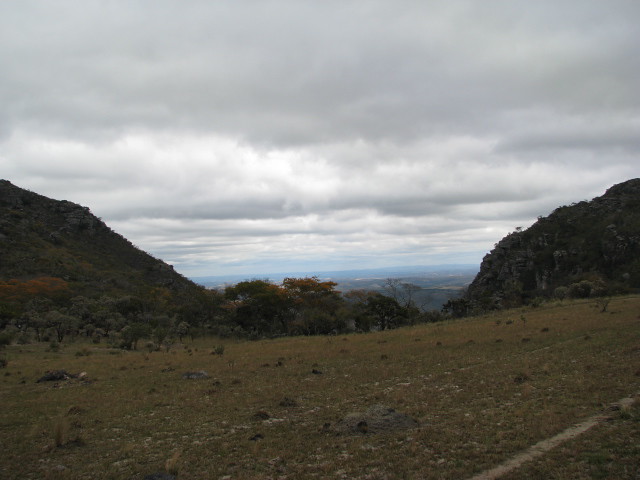This photograph captures a vast mountainous landscape in a landscape orientation, showcasing a serene mountain walkway scene. Dominating the top half of the image is a sky filled with a blend of white and gray clouds, though patches of blue peek through, hinting at a clearing beyond. The photograph is taken from a higher elevation on a flat area with sparse, short grass and small shrubs dotting the foreground. To the left and right of the image stand imposing brown mountains, framing a centrally located gravel or dirt pathway that invites exploration. Extending into the distance, a greenish-brown valley stretches out far beyond where the mountains taper off. The scene creates a picturesque and inviting setting for hiking, with its mix of natural elements meticulously captured in the photograph.